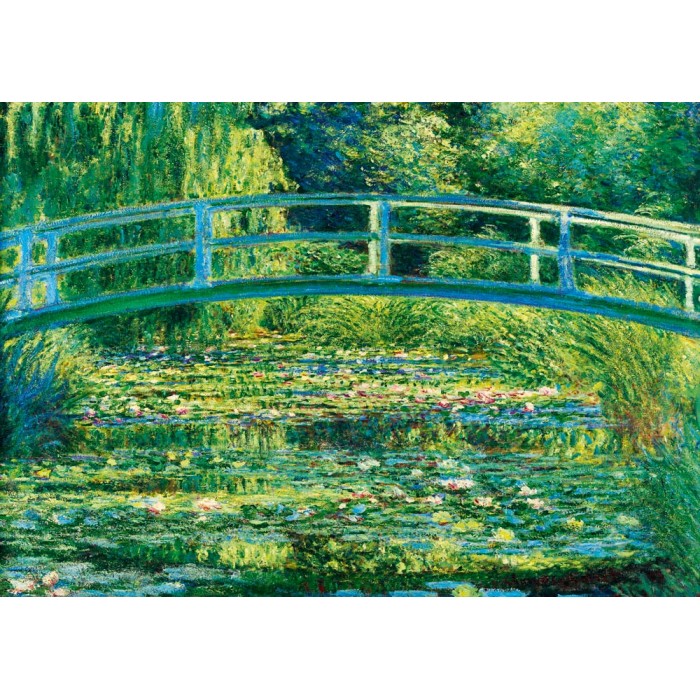This painting, possibly by Claude Monet, captures a serene, vibrant scene dominated by a white arched bridge with two railings, spanning a body of still water filled with numerous lily pads and small white flowers. The bridge, centrally positioned, is surrounded by lush greenery, including shoots of grass, shrubs, and a weeping willow gracefully arching over the water. The water, appearing swampy and moss-covered, is dotted with various water plants. In the background, dense green foliage and large trees create a rich, natural backdrop. The predominant colors in the painting are shades of green and blue, giving the impression of a bright, warm day, evocative of late spring or early summer. The artwork, rendered in a watercolor style, exudes a calm, timeless beauty reminiscent of early 20th-century art.